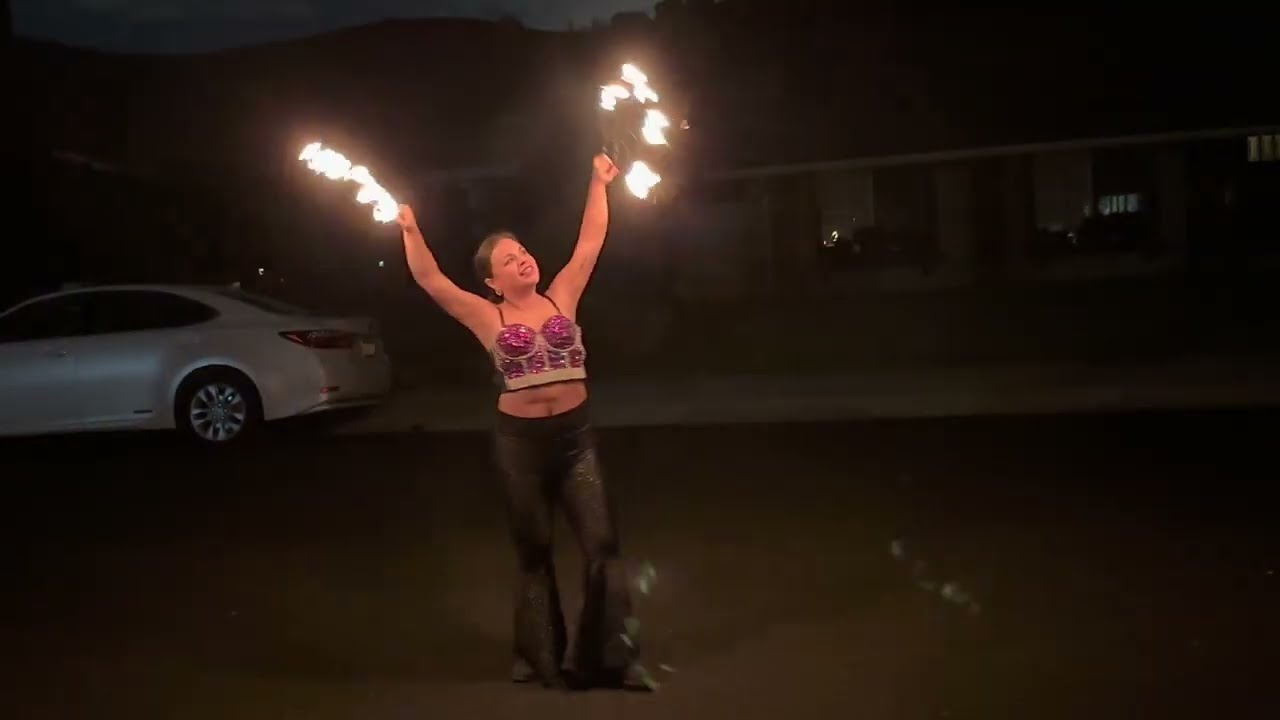In this night-time outdoor scene, a light-skinned Caucasian woman is performing a fire dance, holding rings of fire high in the air. She is dressed in a striking outfit: a costumed bikini top with purple and white glittery accents, exposing her midriff, and tight black bell-bottom pants paired with black boots. Her head is tilted upwards to the right, illuminated by the bright, yellow light of the blazing rings she manipulates. The backdrop features a dark gray, sloped-roof house, with faint light glowing from some of its windows, flanked by a silver sedan to her left. The ground beneath her transitions from a dark gray to a lighter hue closer to the house. The sky, visible in the upper left corner, is a deep, dark blue, completing the vivid night-time tableau.